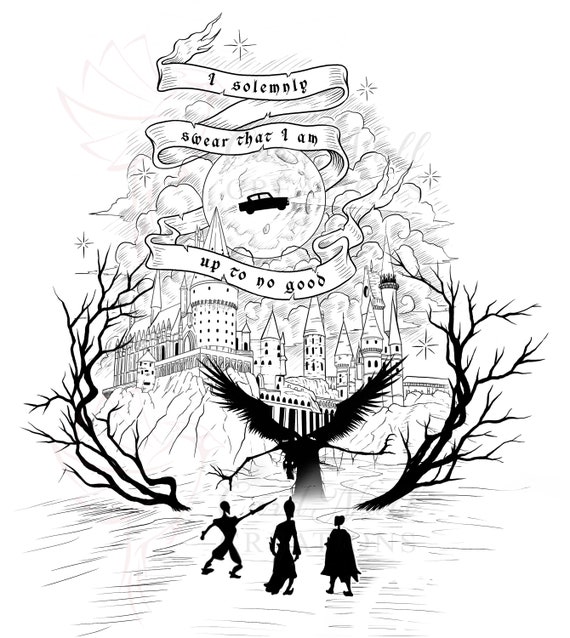This black and light blue digital drawing, designed to look hand-drawn, captures a dark and intriguing Harry Potter scene. At the top of the image, a medieval-style banner with the inscription "I solemnly swear that I am up to no good" drapes across a detailed moon, craters visible, and a silhouette of a flying car with headlights on just below it. Beneath this, Hogwarts Castle with its distinctive parapets and towers perches on a craggy mountain. On either side, stark, leafless tree branches stretch upwards like clawed fingers, drawn in dark black ink. In the foreground, three black silhouetted figures stand with their backs to the viewer, one donning a cape, another appearing to wear a robe or dress, and the third possibly wielding a wand, umbrella, or sword. They're facing a formidable winged creature with spindly long arms and an eerie presence, emphasizing the ominous atmosphere. The entire composition is a monochromatic blend of black with touches of light blue, enhancing its mysterious and magical essence.